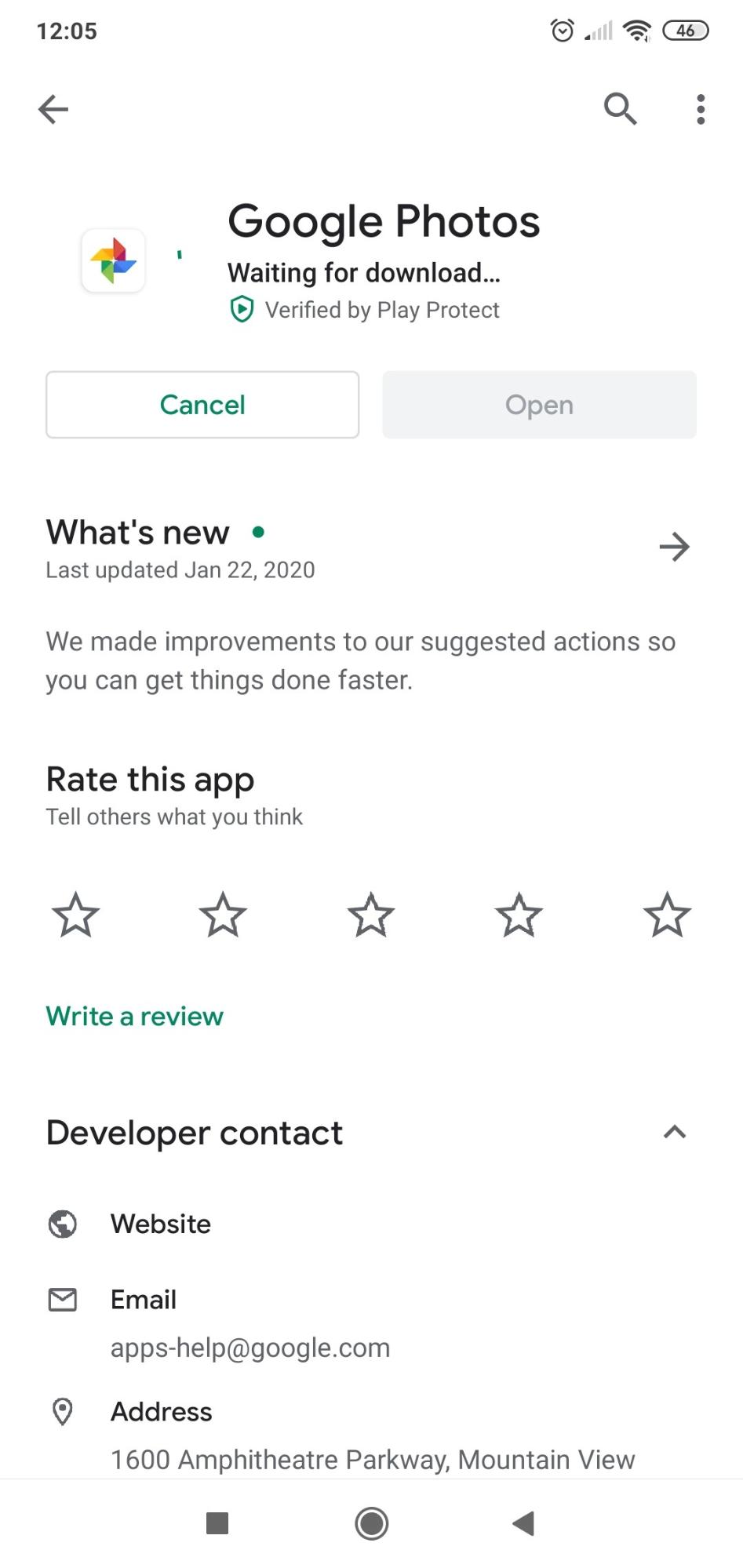### Detailed Caption:

The image showcases the Google Photos application displayed on a smartphone screen. The phone’s status bar is visible, showing the current time, active alarm indicator, Wi-Fi signal strength, cellular signal strength, and a 4G network connection, indicating the phone's model capabilities.

At the top of the screen, there is a search option next to the Google Photos logo. Below it, the display shows a notification stating "Waiting for download" followed by "Verified by Play Protect." Users are presented with two options: "Cancel" or "Open."

Further down, there is a "What's New?" section, dated January 22nd, 2020. The text mentions that improvements have been made to suggested actions within the app to enhance user efficiency.

A prompt also invites users to rate the app, featuring a five-star rating system alongside an option to write a review. For further assistance, there is a "Developer Contact" section listing the developer’s email address (apps/help@google.com) and a physical address at 1600 Amphitheatre Parkway, Mountain View.

At the bottom of the screen, there are three prominent buttons: "Stop," "Record," and "Play," suggesting that the image might have been captured while using a screen recording feature.

Overall, this image provides a comprehensive snapshot of the Google Photos application interface and the additional features and contact details available to users.